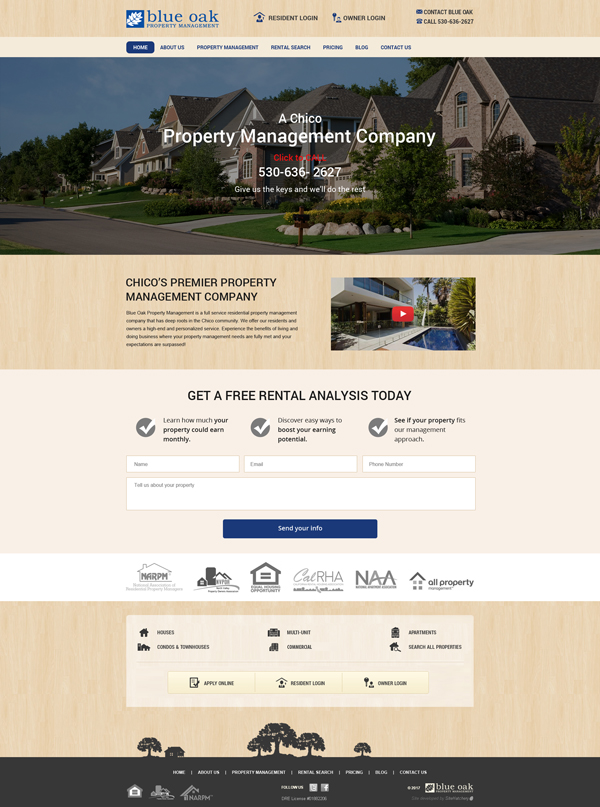This image depicts the homepage of a real estate management firm's website, Blue Oak Property Management. The top section has a beige background and prominently features the company's name, "Blue Oak Property Management," written in blue. Adjacent to the text is a logo consisting of a blue square with a white leaf inside it. Next to the company name are options for "Resident Login" and "Owner Login," followed by a contact number.

Further down, the navigation menu offers several options, including "Home," "About Us," "Property Management," "Rental Search," "Pricing," "Blog," and "Contact Us." Below the menu, a wallpaper image of a picturesque residential street serves as a backdrop for the message, "A Chico Property Management Company. Click to call 530-636-2627. Give us the keys and we'll do the rest."

Beneath this message, there is a brief description of the company's services. It highlights Blue Oak Property Management as "Chico's Premier Property Management Company" and notes that the firm is a full-service residential property management company with deep roots in the Chico community.